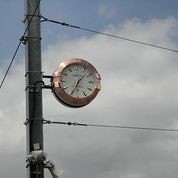A small, detailed photograph captures a street-mounted clock in a daylight scene. Positioned towards the left side of the image, a square column rises perpendicularly, supporting the clock. The clock, framed in a brownish casing, features Roman numerals on a white face with black clock hands, indicating the time as approximately 1:35. Above, a taut support wire angles sharply downward off the left edge of the photo, while two additional support wires extend to the right. In the background, a dramatic cloud bank fills the sky with a sliver of blue peeking through at the top.